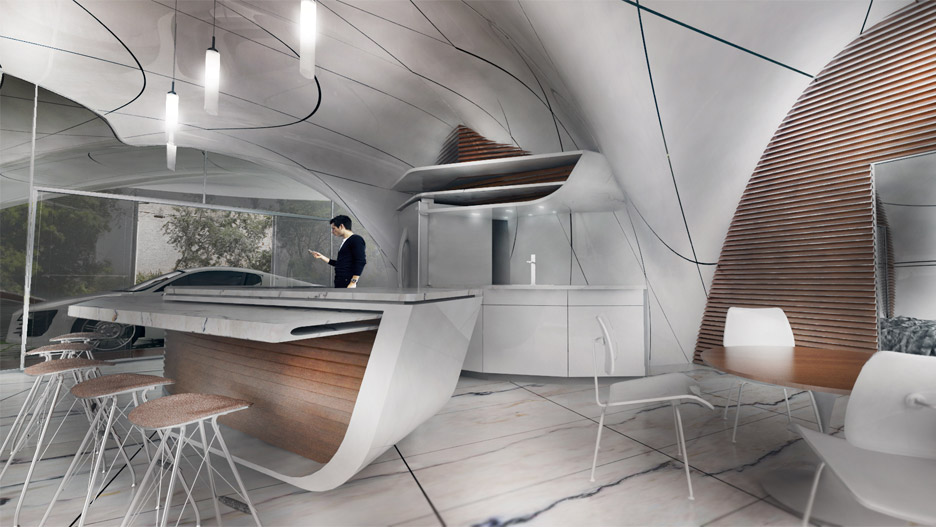The image depicts a highly detailed 3D rendered scene of a futuristic, modern kitchen. Central to the image is a 3D generated man wearing a black shirt, standing near a large window on the center-left side, which offers a glimpse of a sleek white futuristic sports car parked outside. The kitchen's modern aesthetic features a wavy, reflective ceiling and hanging cylindrical lights above a breakfast bar, which is surrounded by stools with wooden seats and white legs. The floor has a minimalistic design with marble and subtle black lines, enhancing the futuristic atmosphere. Behind the man, there are kitchen cabinets, a refrigerator, and a sink, all contributing to the sophisticated and modern appeal of the space. To the lower right, a wooden-top table with white chairs further complements the kitchen's design. The overall color palette leans towards shades of brown, white, and light gray, harmonizing with the modern minimalist theme.